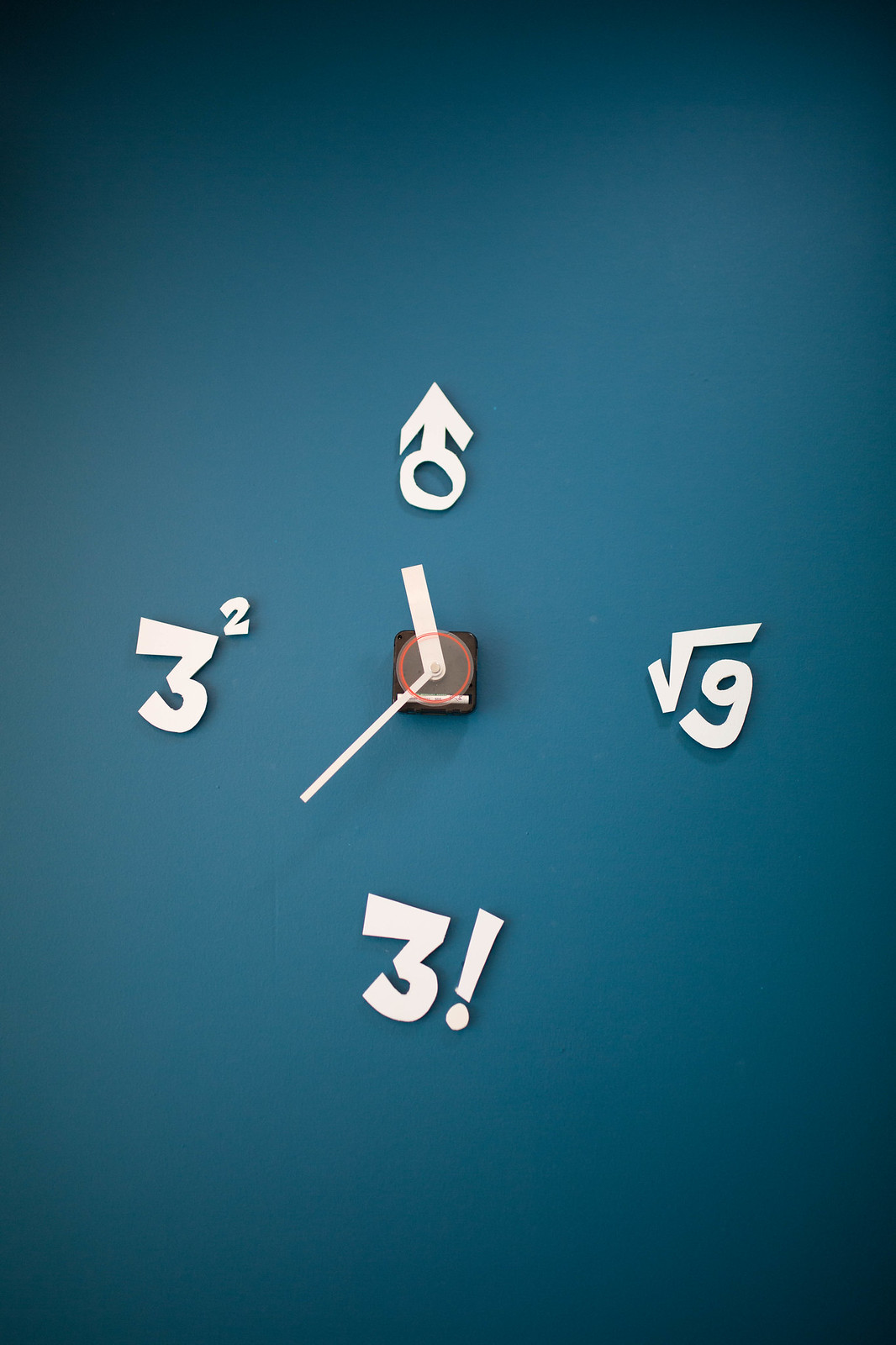The image features a unique mathematician's clock set against a dark teal background that lightens towards the center. The clock, anchored at the center in a black square with a red circle, has two white hands— a short hour hand and a longer minute hand. Traditional numerals are replaced by mathematical symbols: at the 12 o'clock position, there's a white male symbol (a circle with an arrow pointing upwards), at 3 o'clock, the square root of 9 (√9), at 6 o'clock, a 3 followed by an exclamation point (3!), and at 9 o'clock, 3 squared (3²). The overall design creates a visually engaging and intellectually stimulating piece.